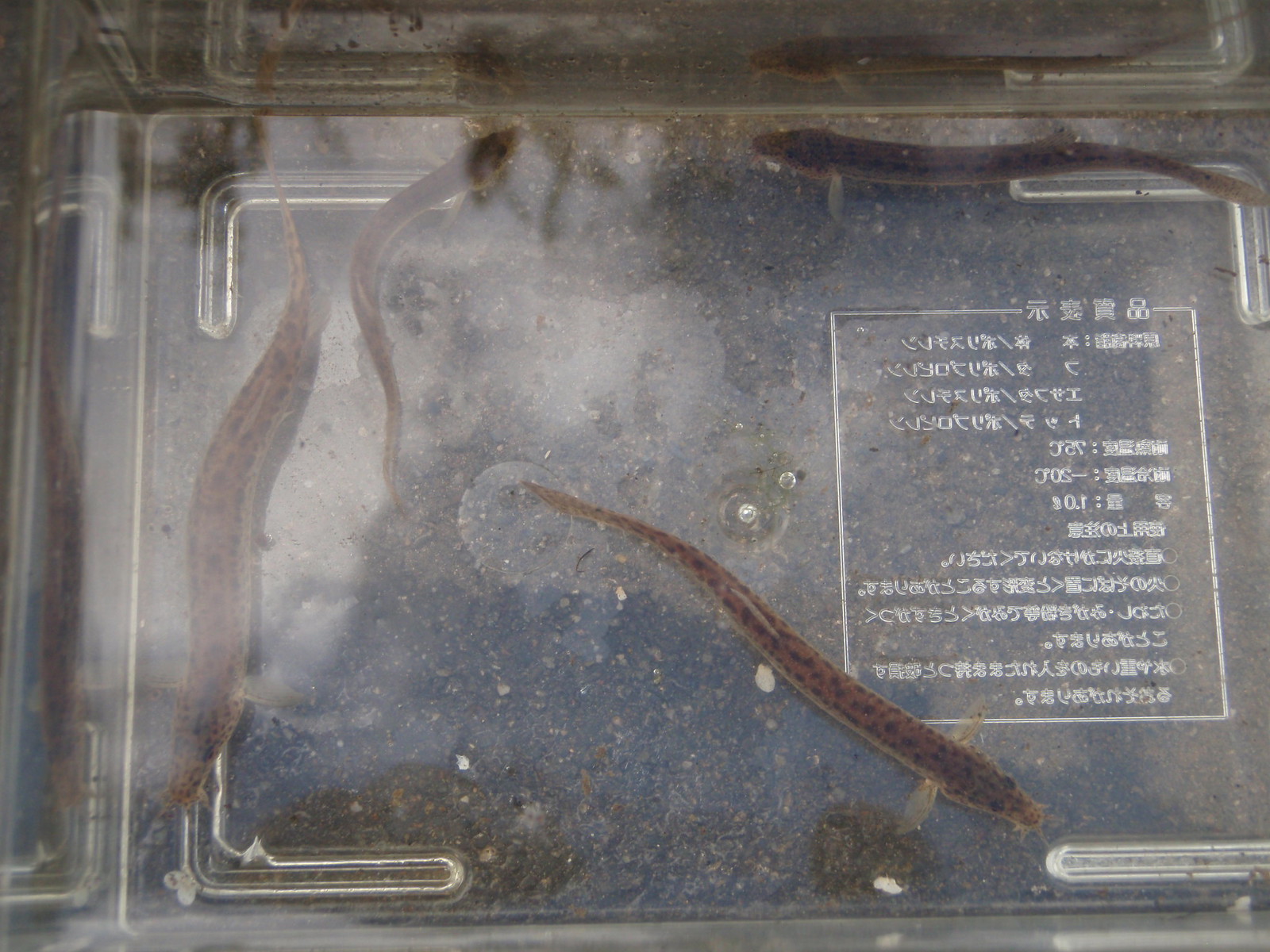This image is an overhead view looking down into a clear plastic or glass container filled with extremely dirty water. Inside the container are four long, slender, tadpole-like salamanders with reddish-brown bodies covered in black spots. The largest salamander is on the left side of the container, positioned with its head towards the bottom and tail reaching almost the top. Near its tail, on the right, is the smallest salamander, wiggling as if swimming, with its head at the top and tail at the bottom. To the right of the smallest one is a medium-sized salamander, with its head facing left towards the small one and its tail on the right side. The second largest salamander is at the bottom, oriented diagonally with its head down towards the bottom right corner and body curving up to the left. These salamanders have flat, light brownish tails, black eyes, and two noticeable gills on their heads. There are four L-shaped raised pieces in each corner of the container, and on the right-hand side, Japanese writing and unfamiliar symbols are visible.